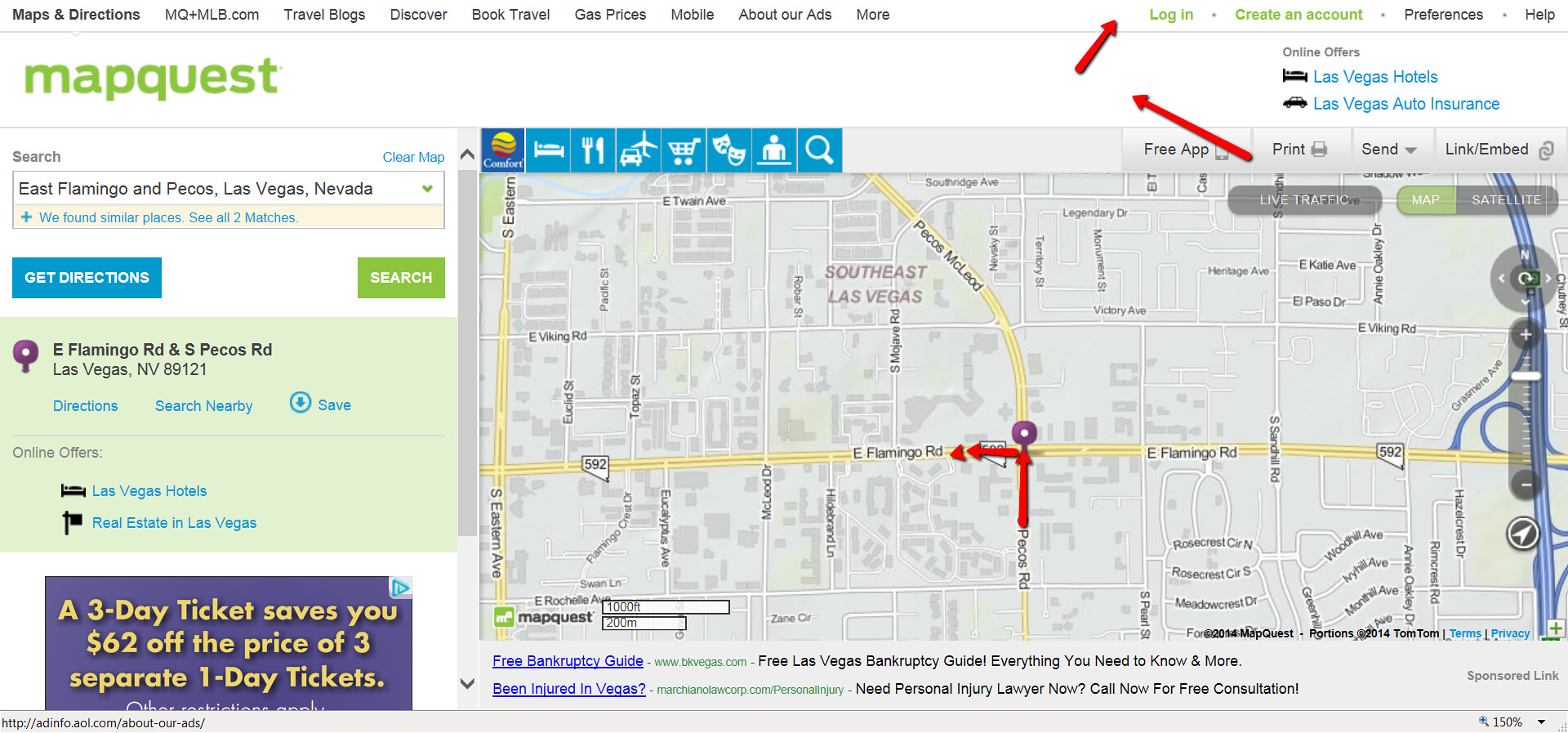A detailed map created using MapQuest, an online mapping service accessible via web and mobile apps, displaying the intersection of East Flamingo Road and Pecos Road in Las Vegas, Nevada. The map prominently features directional arrows in red, indicating the route to the specified destination, which is highlighted with a purple circle. The top section of the map includes an advertisement for a Comfort Inn, featuring icons representing various amenities such as a bed, dining utensils, travel options (plane and car), a theater mask for entertainment, and a frowning face for alerts or concerns. These icons serve as quick links to hotels, restaurants, travel information, and more. Additional map functionalities like 'print', 'send', and 'embed' are available for user convenience. The map layout shows Pecos Road running from north to south and East Flamingo Road running from east to west, along with other nearby streets like Viking Road and Legendary Drive. The detailed visual guide assists users in navigating to the specified location, ensuring they can easily identify and reach their destination using MapQuest services.